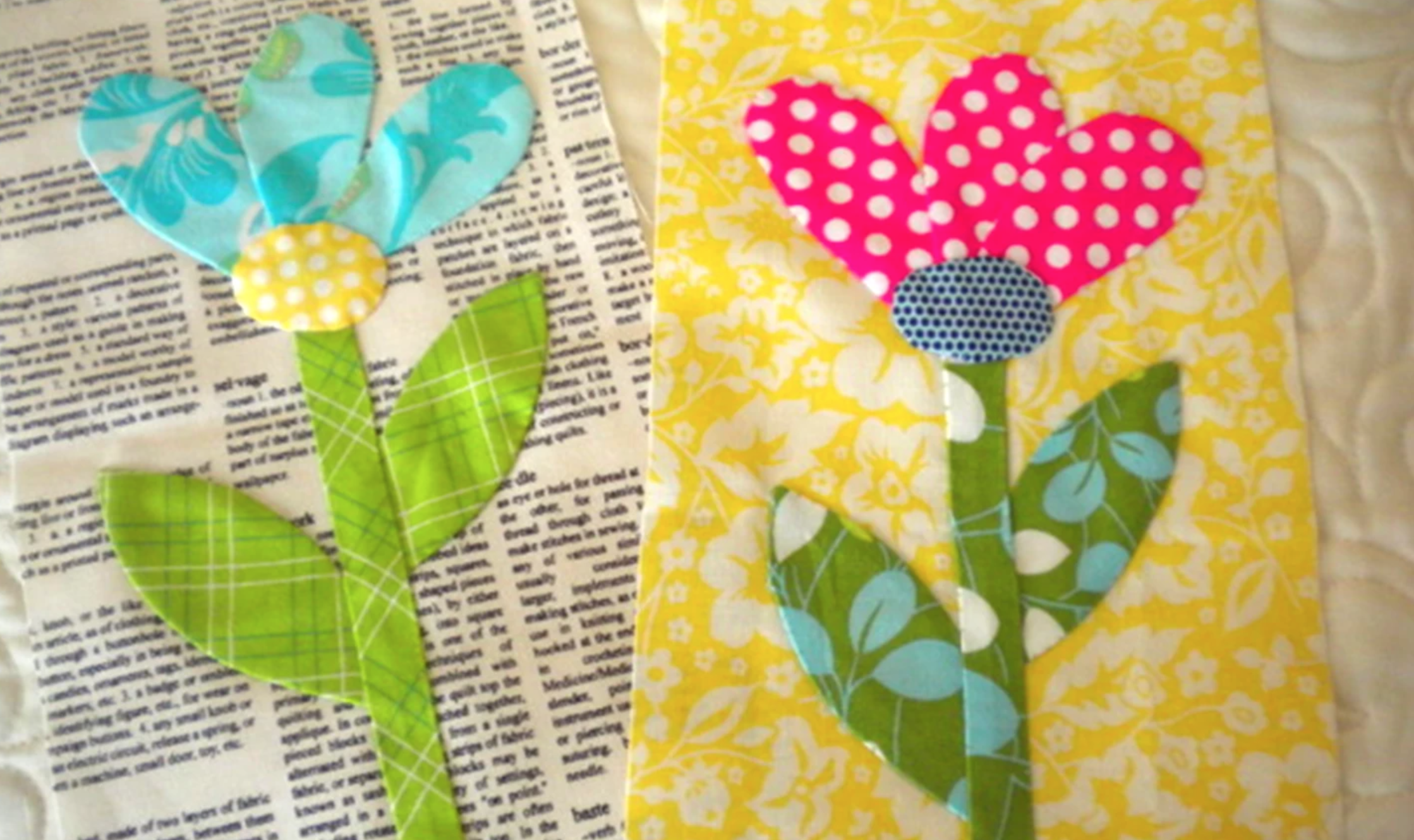This image captures a detailed display of two flower-themed art projects made from various strips of cloth, each showcasing a distinct and vibrant composition. On the left, a flower is set against a backdrop of newsprint. This flower features a green, criss-cross patterned stem and two leaves, also with a green plaid print. Its center is a yellow fabric with white polka dots, from which three blue petals with floral designs emerge.

To the right, the second flower is placed against a yellow and white floral background. This flower has a stem and leaves made from fabric printed with stem and leaf designs. The flower’s center is a blue and white polka dot pattern, while its petals are a striking hot pink fabric adorned with white polka dots. Both art pieces demonstrate intricate craftsmanship and creativity, using a variety of fabric textures and patterns to bring lifelike floral designs to life on contrasting backgrounds.